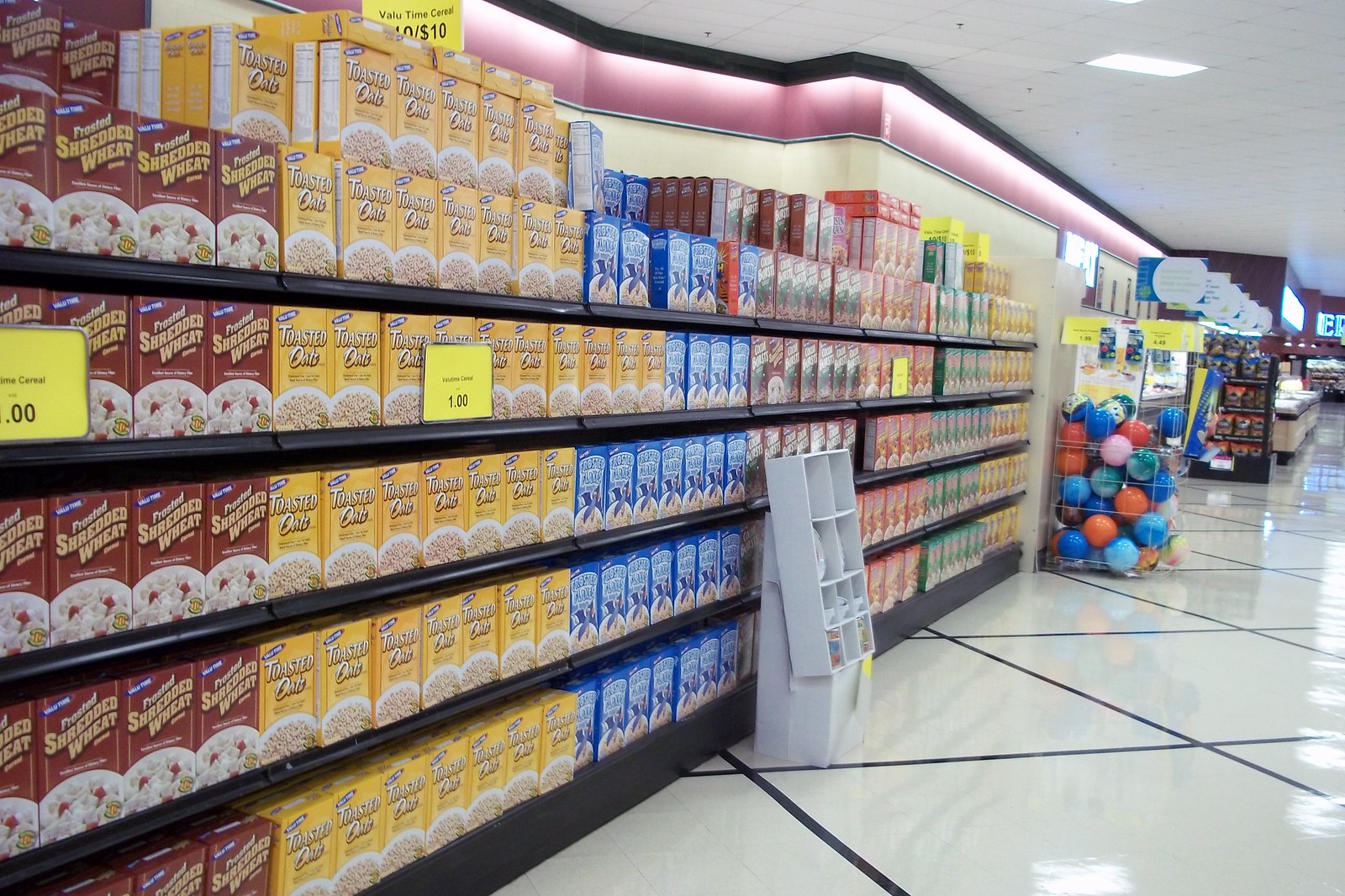The image captures a long, shiny supermarket aisle with large, diamond-shaped white tiles, separated by dark gray grouting, reflecting the white square ceiling lights. The aisle starts with several neat rows of cereal boxes, showcasing different colors: burgundy, yellow, blue, brown, green, and another yellow. Each color-box grouping contains about six boxes per row, with prices visible on yellow tags indicating a charge, though the currency isn't clear. The black shelving unit sits atop a gray border, while just before the brown cereal boxes is a side-view of a white, cardboard display with cutouts that isn't fully visible. Moving further down the aisle, there’s a display of colorful toy balls—blue, red, black, pink—housed in a wire basket. Beyond this, various yellow price signs and indistinguishable displays of brown, white, and light blue items blend into the background, becoming less clear as the aisle stretches into the distance. The ceiling features white tiles with a purple trim and black border near the top of the shelves.